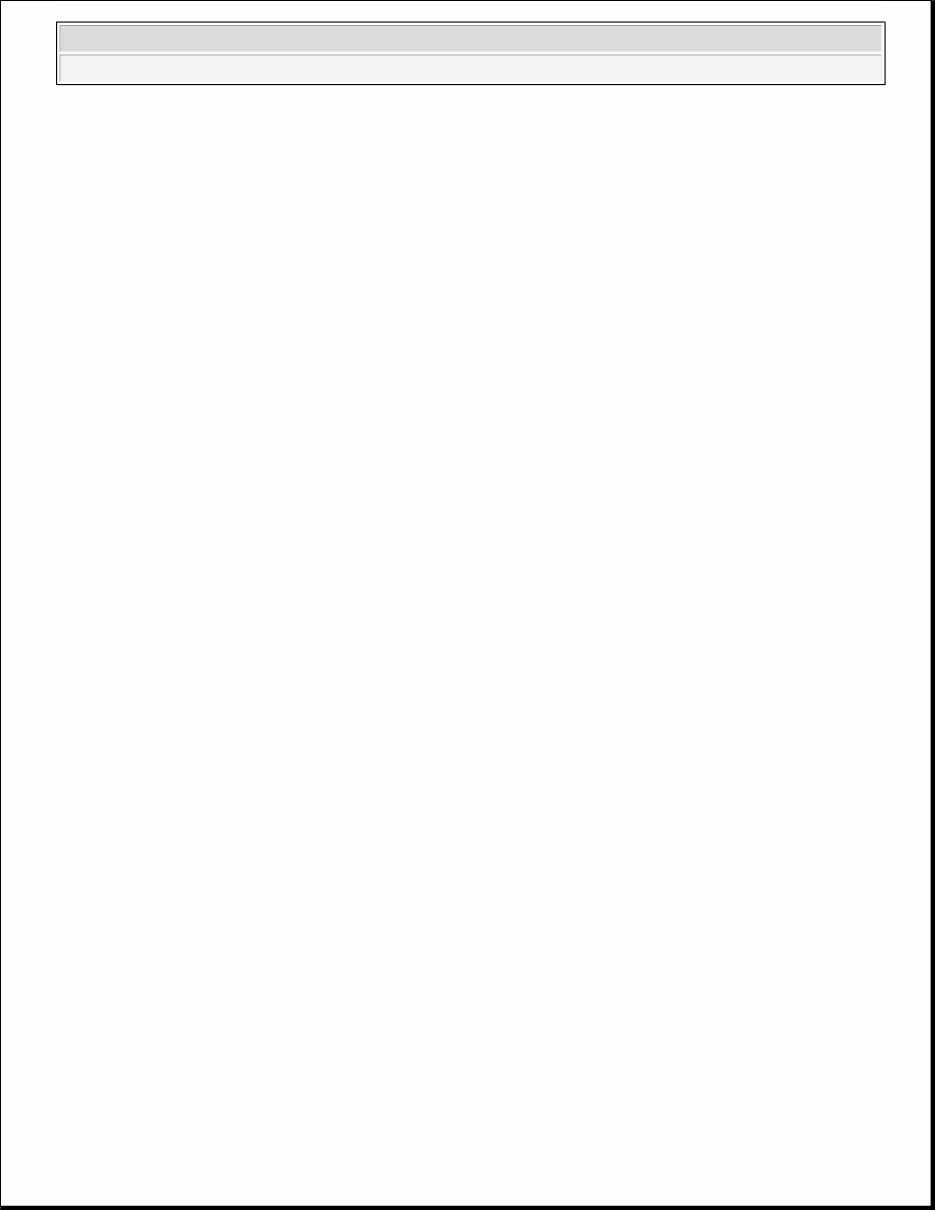The image features a predominantly white background. Along the top edge and left side, there is a light blue line, creating a subtle border. Conversely, the bottom edge and right side are marked by a heavier black line, adding contrast. Centrally placed within this large white expanse is a smaller, rectangular box. This smaller box is defined by a black outline on the left and bottom sides, while the top and right sides are accented with light blue lines, creating a distinctive frame.

Inside the smaller box, the primary color is light blue. Within this light blue space, there exists an even lighter blue line near the bottom edge. Additionally, an area of the box boasts a slightly darker blue hue at the top, transitioning to a very light blue towards the bottom. The overall composition is visually structured with these contrasting and complementing hues of blue and black, creating a layered effect within the central white area. The bottom of the inner box remains blank, adding a sense of simplicity to the intricate design.